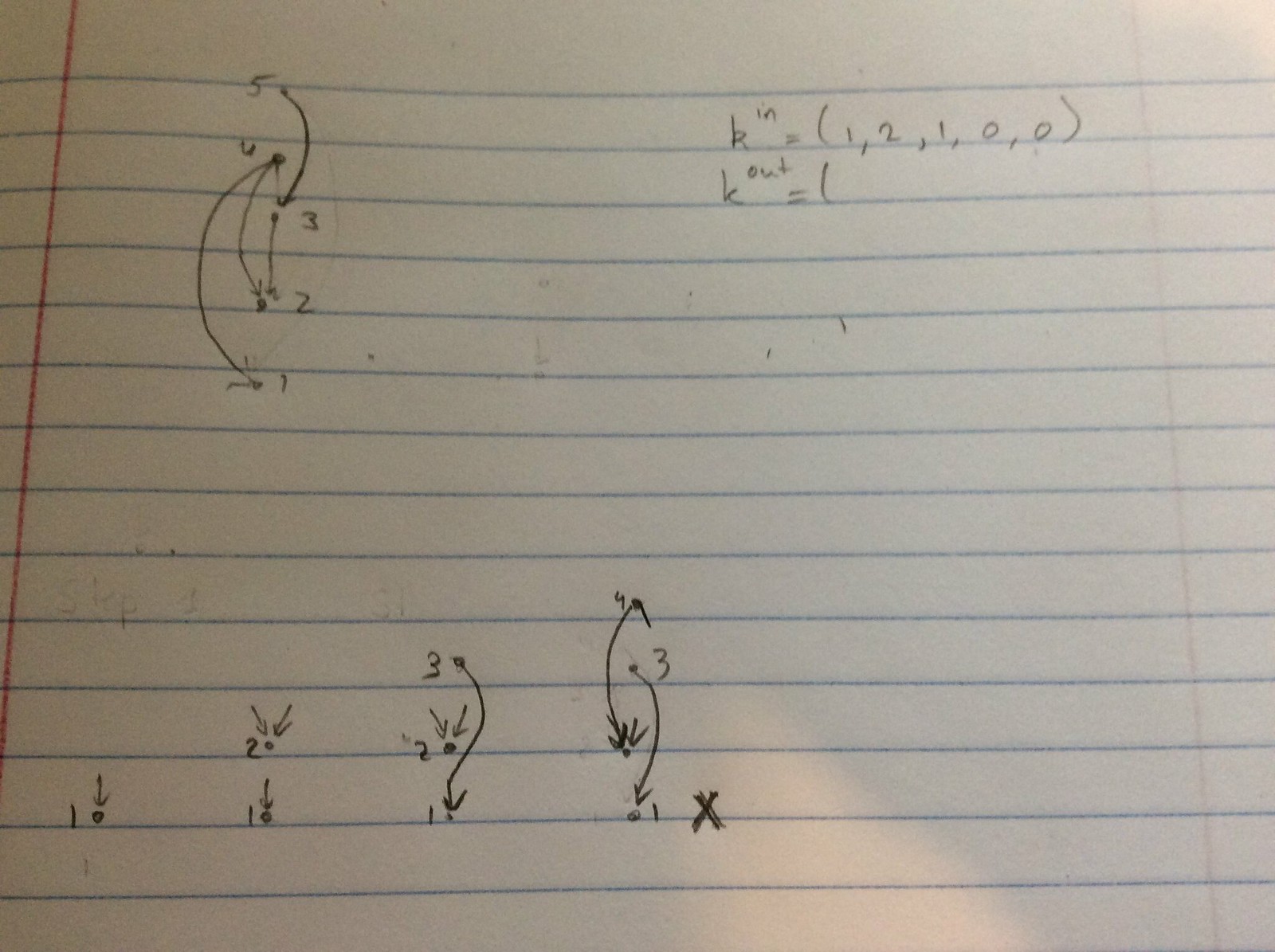Photograph of a piece of lined notebook paper featuring handwritten math problems in pencil. The paper, likely either college-ruled or wide-ruled, is white with the characteristic red vertical margin lines on both the left and right sides and blue horizontal lines. The top-left corner features the number "5" with a dot beside it, connected by an arcing line curving to the right and then back to the left, ending with an arrow and a "3" next to it. From this "3," a segmented line extends downwards to a "2." Further down the initial arc, about two-thirds of the way, is a point labeled "6" from which several vector lines emanate, one going down to a point labeled "2" and another to a point labeled "1."

In the top-right corner of the page, there is a partially visible letter, possibly a "K" or "B," followed by an exponent "N." The equation reads "K^N = (1, 2, 1, 0, 0)." Beneath this, about halfway down the page, the same possibly "K" or "B" appears again but is now written as "K out," with the exponent removed. It reads "K out = ( )."

At the bottom of the page, there is another diagram featuring a "1" with an arrow pointing down to a dot. Below this, a "2" is shown with two arrows pointing to another dot. Beneath this configuration is another arrow pointing to a dot labeled "1."

The detailed mathematical and vector notations on the page suggest complex problem-solving, though the exact meaning of the diagrams and equations remains unclear.